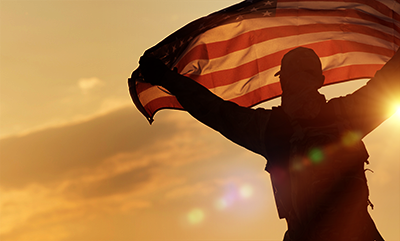In this striking image, a man, likely a soldier based on his heavy clothing and gloves, stands as a majestic silhouette against the backdrop of a vibrant sunset. Positioned slightly to the right, he holds an American flag above his head, with both arms extended in a V formation. The flag appears to catch a gentle breeze, causing it to billow and scoop upwards in the middle, creating a dynamic effect. The vivid sky transitions into a golden amber hue, with patches of golden amber clouds, and a glowing sun peeks partially from the horizon, casting a warm amber light throughout the scene. A noticeable lens flare adds a touch of surreal beauty, emphasizing the setting sun's intense glow. The red and white stripes of the American flag are illuminated by this light, making them glow warmly and adding to the image's patriotic and evocative atmosphere.